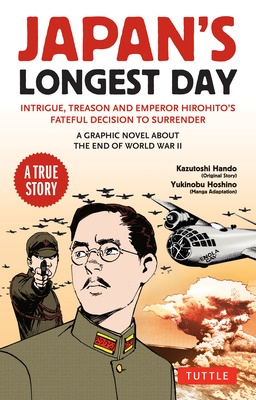This is an image of a book cover titled **"Japan's Longest Day."** At the top, in large capital red letters, it reads **"JAPAN'S,"** with **"Longest Day"** in black letters just below it. Beneath this title, a subtitle in red letters states, **"Intrigue, Treason, and Emperor Hirohito's Fateful Decision to Surrender,"** followed by a smaller caption in black: **"A Graphic Novel About the End of World War II."** On the left side, there is a red seal that reads **"A True Story."** The cover features an animated scene. In the foreground, to the left, there is a man in a military uniform, his body angled slightly towards the viewer, with his face turned towards approximately five o'clock. Behind him, another man is pointing a gun directly at the viewer. In the background, there are several airplanes flying and a large mushroom cloud from an explosion. On the right side under the subtitle, it lists **"Kazutoshi Hando Original Story"** and **"Yutaka Yoshino Manga Adaptation."** At the bottom right corner, there's an emblem that says **"Tuttle."**